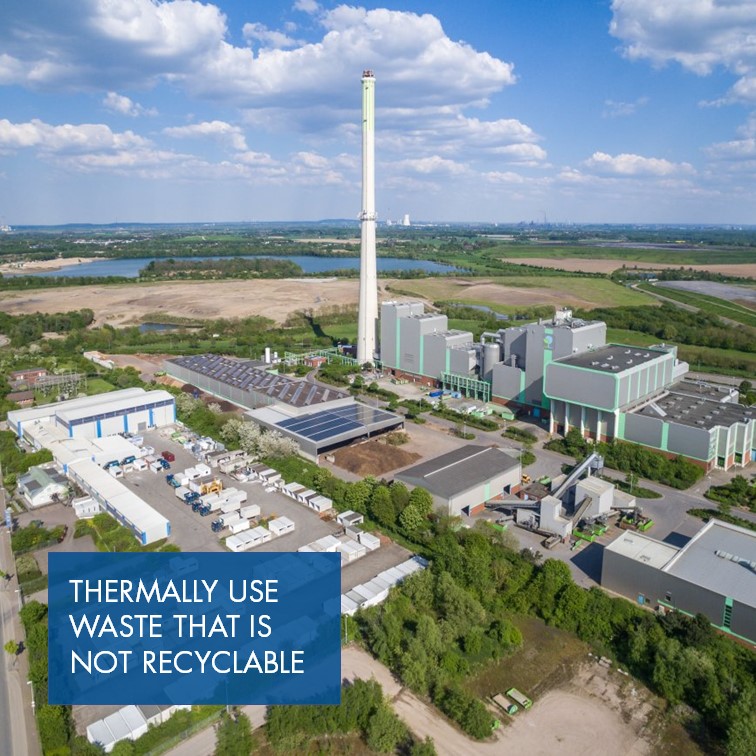This detailed aerial photograph showcases a large, modern industrial complex, prominently featuring a waste processing plant dedicated to thermally using non-recyclable waste. Central to the image is a tall, smoke-free chimney that extends towards the top of the photo, surrounded by a series of interconnected gray buildings of varying heights. Several of these structures are adorned with solar panel arrays, pointing to an integration of renewable energy solutions. The scene also includes numerous white trailers and trucks parked in an orderly manner near warehouse rows and shipping containers, suggesting robust logistical operations.

To the left of the image, conveyor belt machinery hints at the extensive scale of the processing activities within the complex. The industrial buildings are accented with green and blue trims, adding subtle color variations against the dominant gray architecture. Enhancing the image's informative value is a prominent blue text box at the bottom, with white text reading "thermally used waste, that is non-recyclable." Surrounding the facility, green trees dot the landscape, providing a contrast to the man-made structures.

In the background, vast bodies of water and sprawling cityscapes stretch out towards a horizon marked by a distant power plant, characterized by a tall, white smokestack. The expansive and flat terrain under a blue, lightly cloudy sky adds depth to the photograph, highlighting both the industrial prowess and the environmental context of the region.